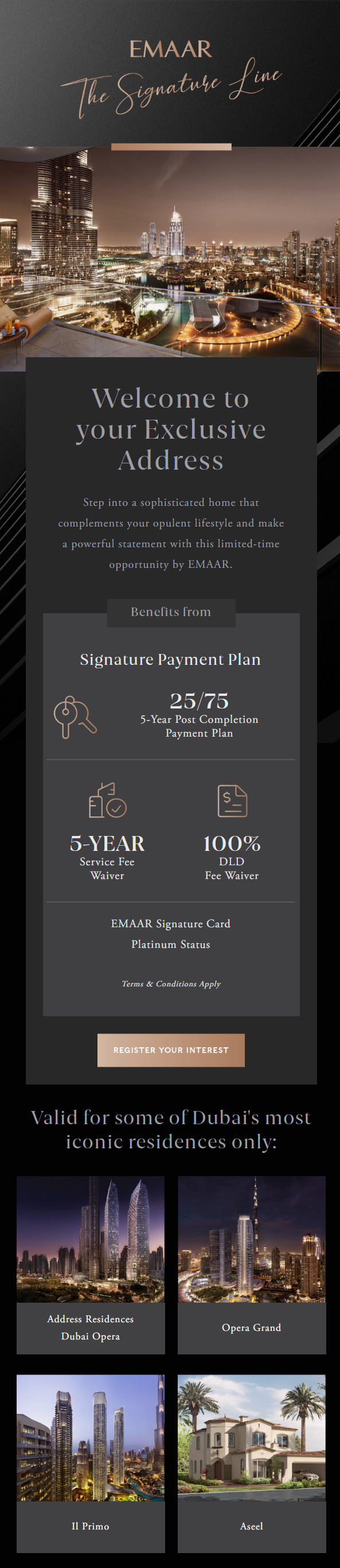The image appears to be a promotional webpage from a real estate website, featuring a sophisticated design and high-end offers. 

At the top, there's a black border with "EMAR" displayed in gold, uppercase letters. Below it, the phrase "The Signature Love" is elegantly written in cursive. Under this header, a cityscape is depicted with a deep purplish-black sky, featuring skyscrapers and high-rises prominently on the left, with various other buildings and illuminated bridges possibly depicting highways.

Further down, a black box with white text reads, "Welcome to your exclusive address." Additional text within this box is partially legible, mentioning a "powerful statement" and something about a "limited appointment by EMAR."

A black tab with the word "Benefits" in white, uppercase letters, opens up into a lighter black box containing white text that outlines several key features:
- "Signature Payment Plan 25-75" possibly referring to a two-year post-completion payment plan, with a gold outline of keys to the left.
- A gold checkmark icon next to text stating a "Five-Year Service Fee Waiver."
- An icon of a document with a dollar sign, indicating a "100% Old Fee Waiver."
- "EMAR Signature Card Platinum Status" with terms and conditions applying, displayed in white text at the bottom.

An orange box with white text prompts users to "Register Your Interest," followed by white text stating that the offer is valid for some of Dubai's most iconic residences only. 

Below are four locations, each with a brief description and a visual:
1. The first location features two striking glass buildings against a purple sky, partially readable as "Address..."
2. The second is possibly labeled "Opera Grand," showing a single glass building.
3. The third location name looks like "Prime" or "Primo," with an illustration of three high-rises.
4. The last location appears to show a large, two-story single-family residence with an unreadable name starting with an "A."